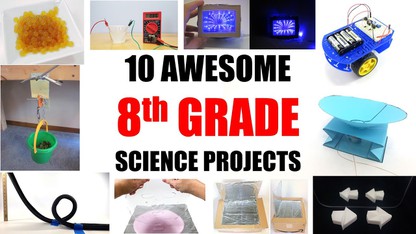The image is a promotional flyer titled "10 Awesome 8th Grade Science Projects" against a white background. The text is centrally placed, with "10 Awesome" in bold black font, "8th Grade" in red, and "Science Projects" also in black. Surrounding the central text are numerous smaller photographs illustrating various science project ideas. 

In the top left corner, there's an image of a white container filled with yellow, wet-looking beads resembling Orbeez. Adjacent to this is a black and red battery pack with protruding red and black wires. Continuing right, there are two pictures featuring blue screens possibly illustrating electrical or digital experiments, followed by a blue battery-powered vehicle with black tires and glowing blue lights. 

On the top right, there's a blue car with yellow-rimmed wheels and visible batteries. Just below it, a light blue object sits atop a dark blue box. Below this, a black box with white arrows pointing in multiple directions is seen. 

In the bottom right, an image displays a green bucket hanging from an apparatus, potentially for a weight or pulley experiment. Next to the bucket, there is a collection of black wires, some tinfoil, and white arrows on a black background. Moving left, different images showcase items such as a glass of water with red and green cords beside it and hands dripping water onto a pink surface framed by a gray square.

The varied photos on the flyer display a rich palette of colors including gold, green, black, pink, brown, pale blue, yellow, and dark blue, capturing the diverse and creative nature of the science projects.